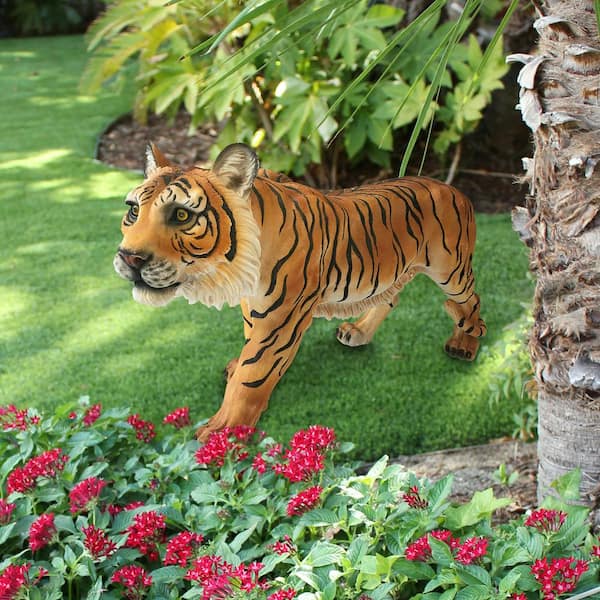This vibrant color photograph captures a picturesque garden scene centered around a striking tiger figure. The tiger, which appears to be either a meticulously photoshopped drawing or a statue, is the focal point of the image. Exhibiting the characteristic orange hue with black stripes, the tiger features a white beard, underbelly, and ear interiors. Its piercing yellow eyes gaze to the left, while its body stretches to the right, standing majestically on a lush green lawn. Below the tiger, vibrant red flowers add a splash of color, enhancing the garden's beauty. To the right edge of the photograph, a tree trunk is partially visible, framed by a mix of greenery and foliage in the background. The lawn extends upwards to the upper left corner, bordered by dense shrubs that complete this serene garden composition.